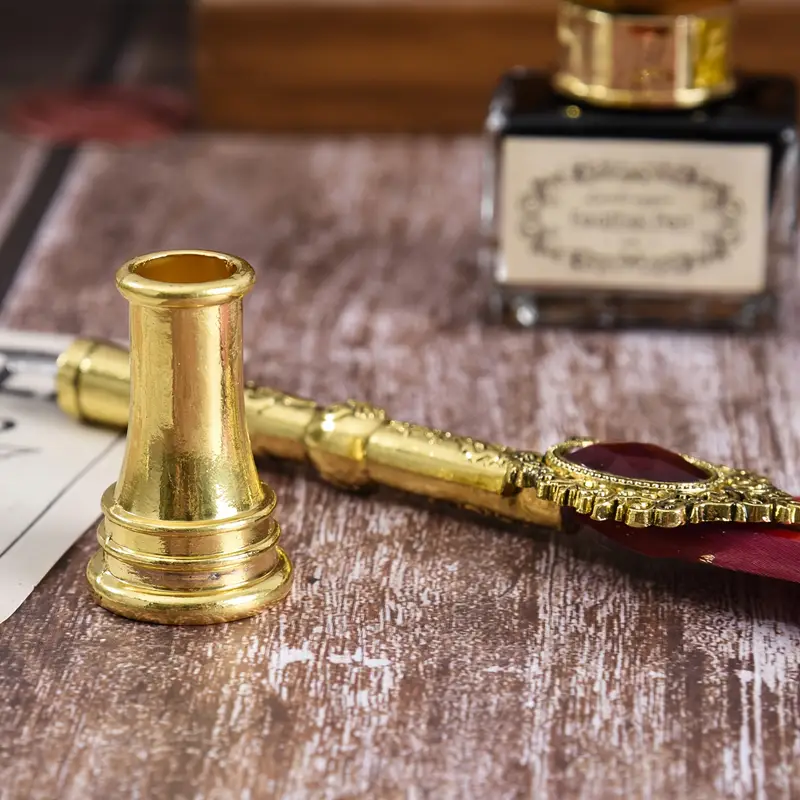The image, a square-format color photograph, exhibits a detailed and realistic portrayal of a brass-colored spyglass with intricate design elements. The spyglass, positioned at an angle with its lower end on the right side of the frame, dominates the center of the image. It is notable for its ornate detailing, including a red gemstone set within a golden frame near its right end and a dark burgundy top with a jewel-like effect.

Accompanying the spyglass is a fluted, cylindrical piece, wider at the base than the top, with a small rim at its opening. This piece, also brass in color, is positioned in front of the spyglass and appears to attach to one of its ends. The items rest on a weathered brown wooden surface, marked by numerous white streaks where the wood's finish has peeled away.

In the background, slightly out of focus on the upper right, is an additional golden object resembling a small trophy, placed on a glass platform. A brown object, mostly obscured, is also discernible in the background. The composition and style of the photograph emphasize a realistic representation, drawing attention to the intricate details and textures of the objects.